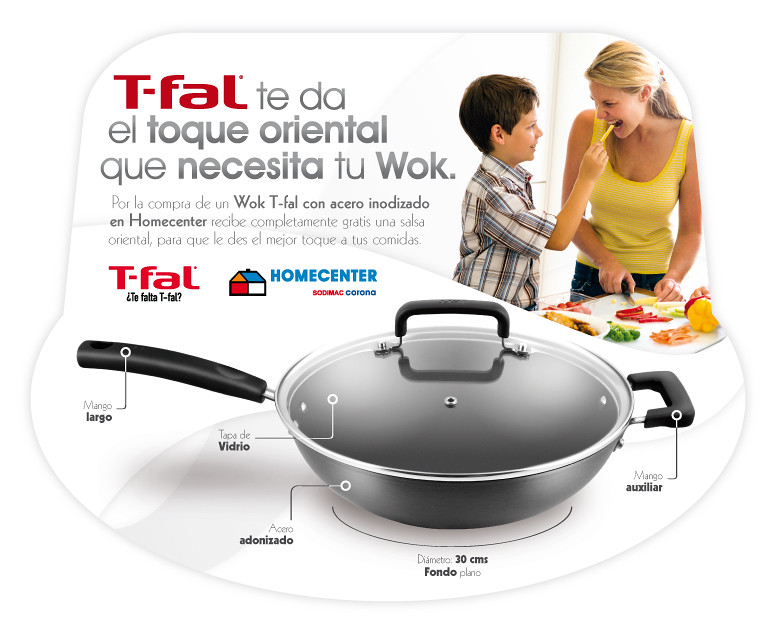This advertisement features a highly detailed image for a Tefal cooking wok, with prominent branding and description in Spanish. The advertisement displays a curved design, wider at the base with no sharp edges, likely designed to sit in the bottom of the wok's packaging. The top section showcases a vibrant scene of a smiling blonde woman with her hair in a ponytail, wearing a yellow tank top and blue jeans, preparing a meal with her young son. The son, clad in a beige plaid shirt with maroon, white, dark blue, red, and black stripes, is joyfully feeding her a piece of yellow pepper. Surrounding them are various fresh vegetables including red and orange peppers, carrots, celery, broccoli, and cherry tomatoes in a plastic container. To their left, there appears to be a bowl of either chicken or breaded food.

Below this heartwarming scene, the focus shifts to the Tefal wok itself, detailed in brushed silver with a dark gray non-stick coating and black handles. The wok's design features a clear glass lid with a steam vent, secured by two silver rivets and a curved black handle. The ad also highlights specifics such as the wok’s dimensions (30 cm diameter), flat bottom (Fondo Plano), and additional side handle (Mango Auxiliar). The Home Center logo, depicted in multiple colors—blue, red, orange, and white—alongside the Tefal branding, punctuates the visual, aligning with the functional beauty of the wok and the joyful cooking experience it promotes.